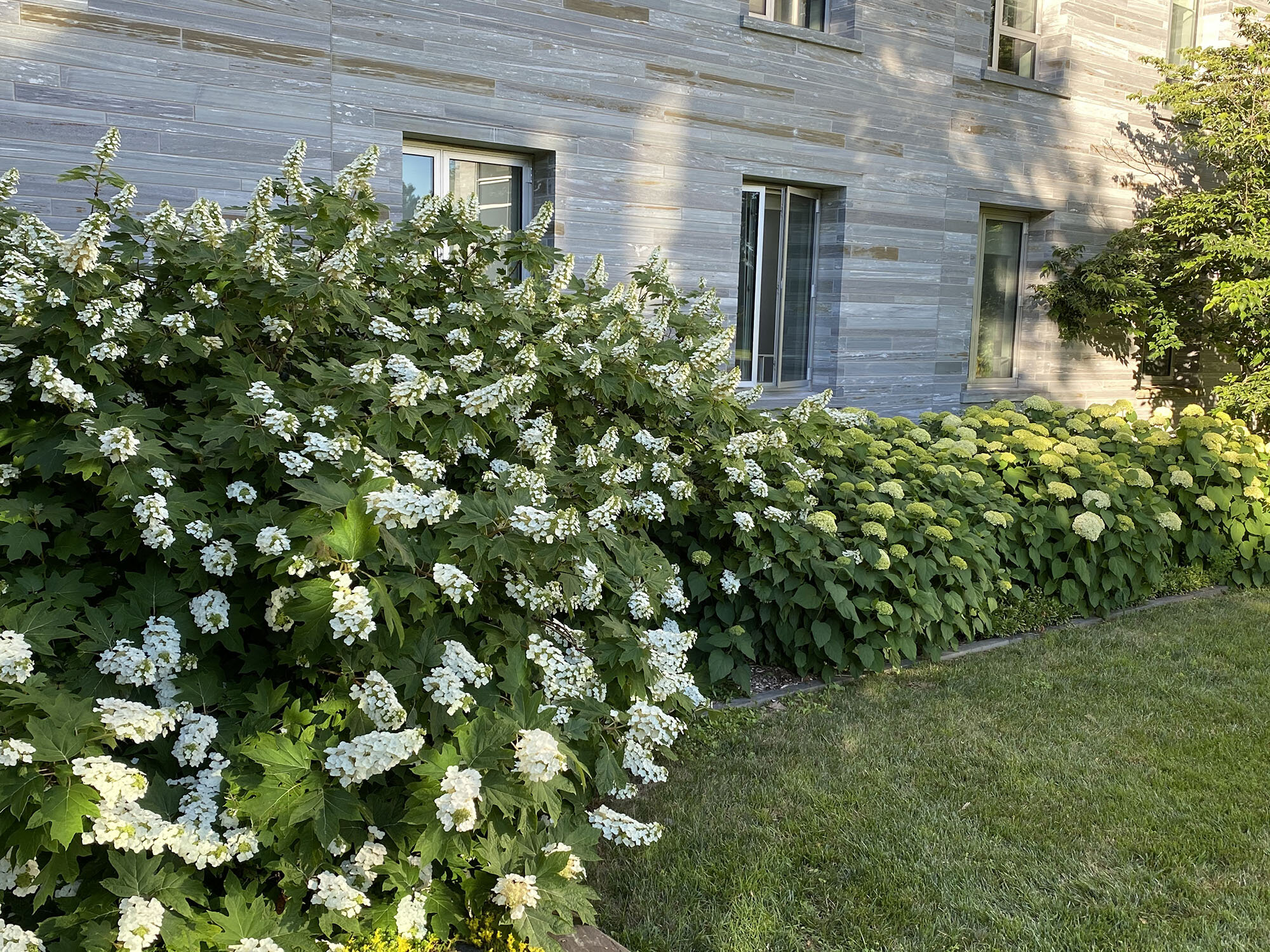This photograph captures a multi-story building with wooden side paneling in shades of grey and brown, showcasing a lush garden in the foreground. The lower part of the structure reveals four windows per floor, with only the lower set fully visible and the upper ones partially cropped out. Prominently displayed in front of the building are expansive, green flowering bushes, adorned with clusters of white flowers. These bushes stretch along the side of the structure and are interspersed with some varieties that have wider leaves—likely hydrangeas—with yellowish flowers amidst the predominant white. The well-trimmed grass beneath these bushes complements the verdant landscape. On the right side of the image, a large, leafy tree partially enters the frame, adding to the rich foliage. The precise and orderly garden creates a serene and aesthetically pleasing scene, highlighting both the natural beauty and the architectural elements of the building.